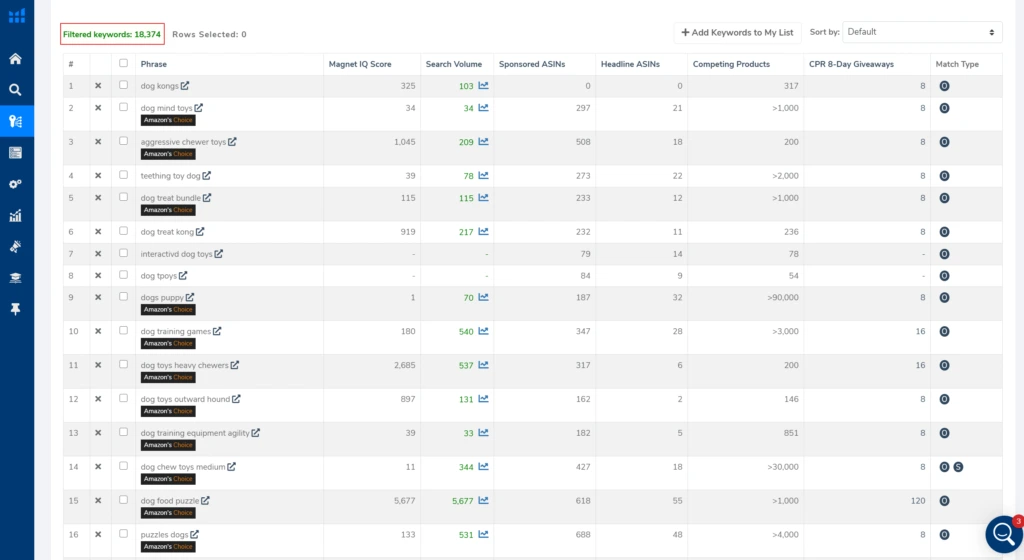Screenshot of a Keyword Checklist Interface:

The image is a screenshot of a keyword checklist interface featuring a white background with structured data presented in alternating rows of gray and white. On the very left side, there is a vertical blue column featuring various icons: a home icon, a search symbol, a key, a square, a bar graph, a thumbtack, and four more unidentified icons.

At the top of the chart, there is a title that reads "Filtered Keywords: 18,374" with an annotation below it stating "Row Selected: 0." Below this title is an action bar with two primary options: a button labeled "+ Add Keywords to My List" and a dropdown menu to "Sort by Default."

The main content displays a list of 15 entries related to keywords. Each entry comprises multiple columns with different types of data: a phrase, a Magnet IQ Score, Speech Volume Measurement, Sponsored ASINs, Headline ASINs, Competing Products, and CPR 8-Day Giveaways.

This detailed layout appears to assist users in managing and analyzing keyword data effectively, providing various metrics and sorting options to enhance keyword selection and prioritization.